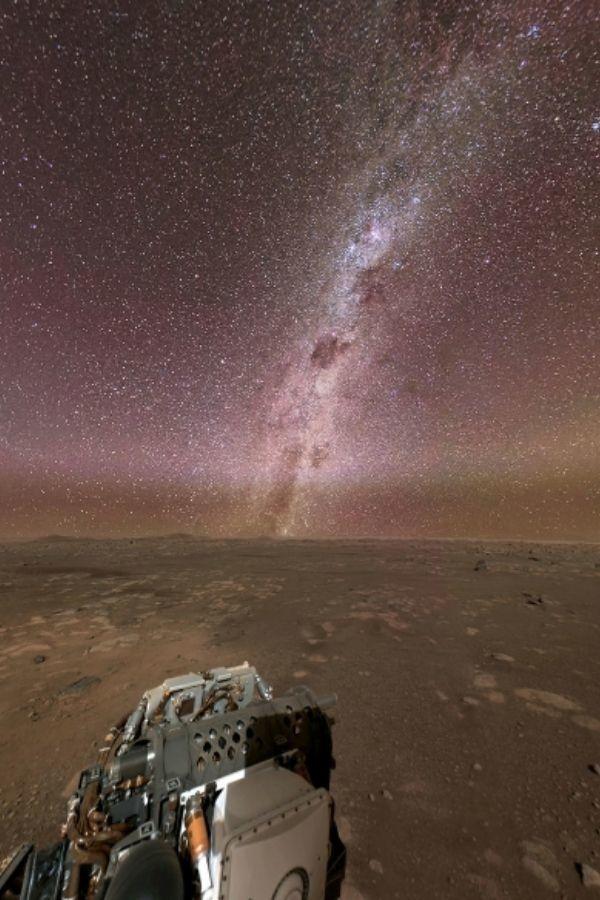In the image, taken by what appears to be the Mars rover, we observe a desolate, brown and gray surface extending across the bottom half of the photo, marked by small craters and pockmarks. A piece of machinery, primarily white and gray with touches of orange and some black details, is positioned prominently in the bottom left, showcasing its metallic and somewhat plastic appearance. The night sky dominates the upper portion of the image, displaying a vibrant array of stars. These stars, in varying shades of white and blue, are particularly dense in a stripe resembling the Milky Way, stretching from the center towards the top right corner. The sky itself transitions from a dark near-black at the top to purples and pinks near the horizon, contributing to a surreal, otherworldly backdrop devoid of any text.